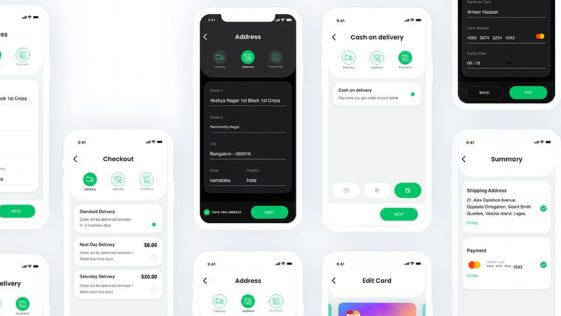Here is a cleaned-up and detailed caption for the image:

"The image consists of multiple phone screenshots organized in five vertical columns. Starting from the left, the first column contains a half and an eighth of a screenshot. The second column has five screenshots: one showing the right half of a screen, followed by an upper corner of another screen. Below these, there is the top two-thirds of a screen, a full screenshot, and lastly, just the top portion of another screen. The third column features a full screen and an additional full screen with only the top portion visible below it. The fourth column displays the bottom half of a screen and then the top three-quarters of another screen. In the fifth column, the top screen is black, and immediately below it, a full screen with a black background is visible. All other screens have white backgrounds. The content within the screenshots includes a checkout page, cash-on-delivery options, address details, an edit card screen, and a summary, indicating various stages of an app's user interface, likely for an e-commerce application."